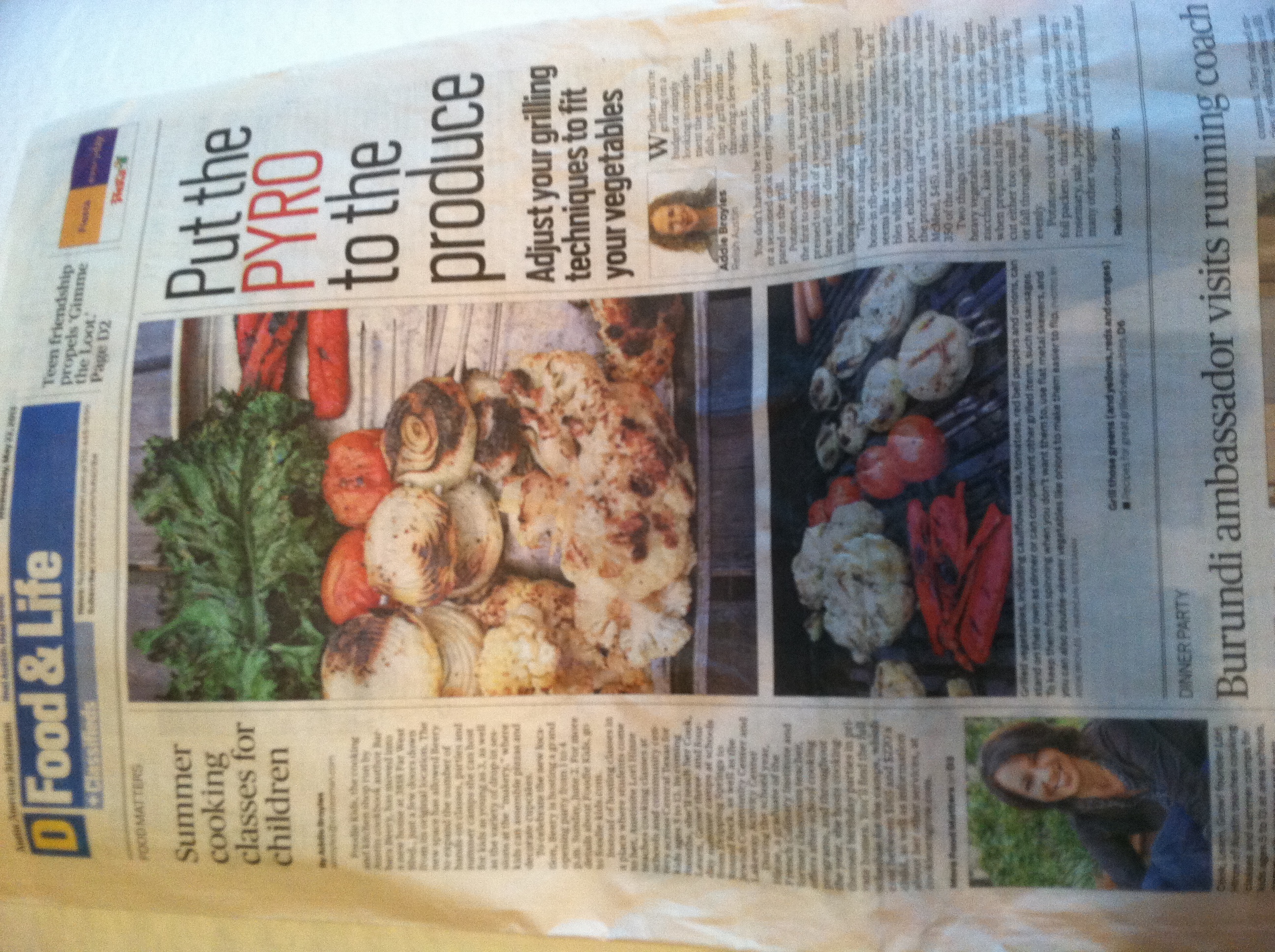The image depicts a horizontally oriented newspaper or magazine section titled "Food and Life," prominently displayed in white text within a blue box at the top left. This section, dedicated to lifestyle and cooking, features multiple articles centered around culinary topics. The newspaper has been rotated 90 degrees counterclockwise, with the top of the page appearing on the left side of the screen and the bottom on the right.

On the left-hand side, a vertical column titled "Summer Cooking Classes for Children" is present, detailing opportunities for kids to learn cooking skills during the summer. The main focus of the page is an article titled "Put the Pyro to the Produce," with the word "Pyro" highlighted in red, suggesting a discussion about grilling or cooking produce with fire. Supporting this theme, the center of the image showcases a variety of grilled vegetables including white and brown mushrooms, red tomatoes, and leafy greens such as spinach, displayed on a grill.

On the bottom left, there is a photograph of a woman wearing a black shirt and holding a blue bag, likely one of the authors contributing to the section. The newspaper then transitions to other news content on the right side of the image, with a headline reading "Burundi Ambassador Visits Running Coach," signifying the end of the "Food and Life" section and the continuation of broader news coverage.